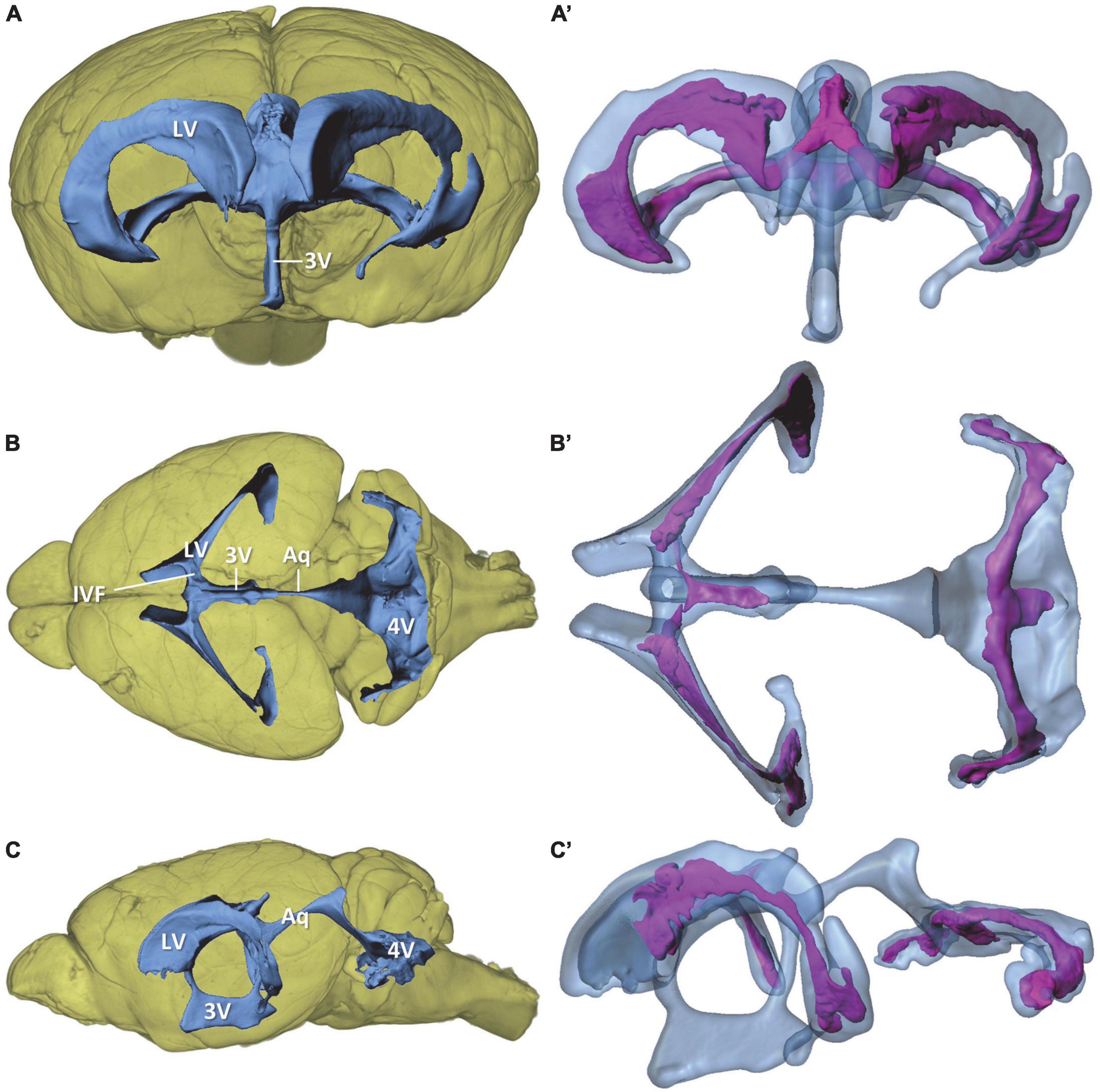The image depicts a detailed scientific poster, likely intended for display in a science classroom. It showcases a 3D computer-generated model of what appears to be a make-believe brain or a unique creature's head structure. The poster is organized into two columns and three rows, labeled A, B, and C. Each row consists of a pair of images: on the left (A, B, and C) are depictions of the brain structure surrounded by tissue, including cutaway versions to show the internal details. On the right (A', B', and C') are the corresponding views of just the bone structures, colored blue with purplish veins inside. The images present different perspectives: A and A' are head-on views, B and B' offer overhead views, while C and C' provide side views. The bones appear spliced and highlighted in gray, blue, and purple to illustrate intricate internal features.